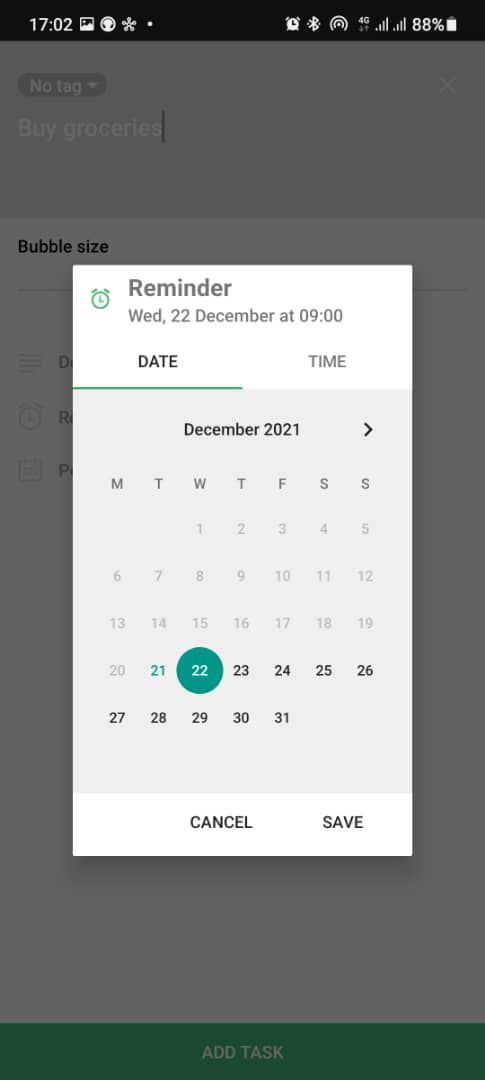A close-up screenshot from a smartphone displays the digital calendar for the month of December 2021. The dates "21" and "22" are highlighted in green, with the 22nd circled in green. The screen also shows it's 17:02, with various icons, including a flower, at the top. The battery indicator on the right shows an 88% charge. Below, a note reads “no tag, buy groceries.” Toward the bottom, there's an entry labeled "Reminder" with a clock icon beside "Wed 22 December at nine o'clock." At the very bottom, large black letters spell out "CANCEL" and "SAVE" in all capitals. The background of the calendar is a soft gray, and there is a prominent green button labeled "ADD TASK."